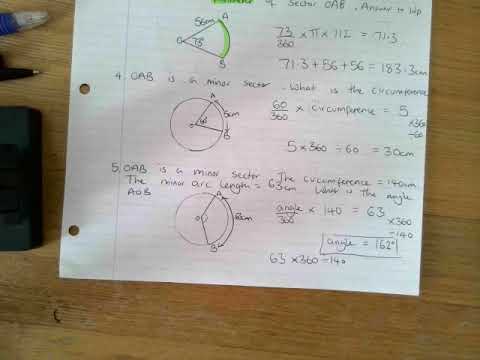The image displays a single sheet of white notebook paper with horizontal lines, featuring three-hole punches along its left margin. The paper, centered on a light brown wooden desk with visible wood grain, is adorned with various mathematical equations and geometric drawings. Predominantly, there are illustrations of a circle with segments removed, radii, and points labeled with letters such as A and B. Mathematical notations are interspersed among the sketches, although they are partially obscured and difficult to decipher. The writing on the paper is primarily in black ink, with occasional lime green highlights.

Positioned to the left of the sheet are several writing utensils, including an open black pen, a second pen with a silver tip and blue accent, and possibly a pencil. Beneath these writing tools lies a black rectangular object, which could be a calculator, an eraser, or potentially a USB stick, due to its indistinct, shadowy appearance. Despite the cropped view, a sense of order suggests someone is diligently working through mathematical problems, likely geometry, with numbers and formulas scattered across the paper's surface.